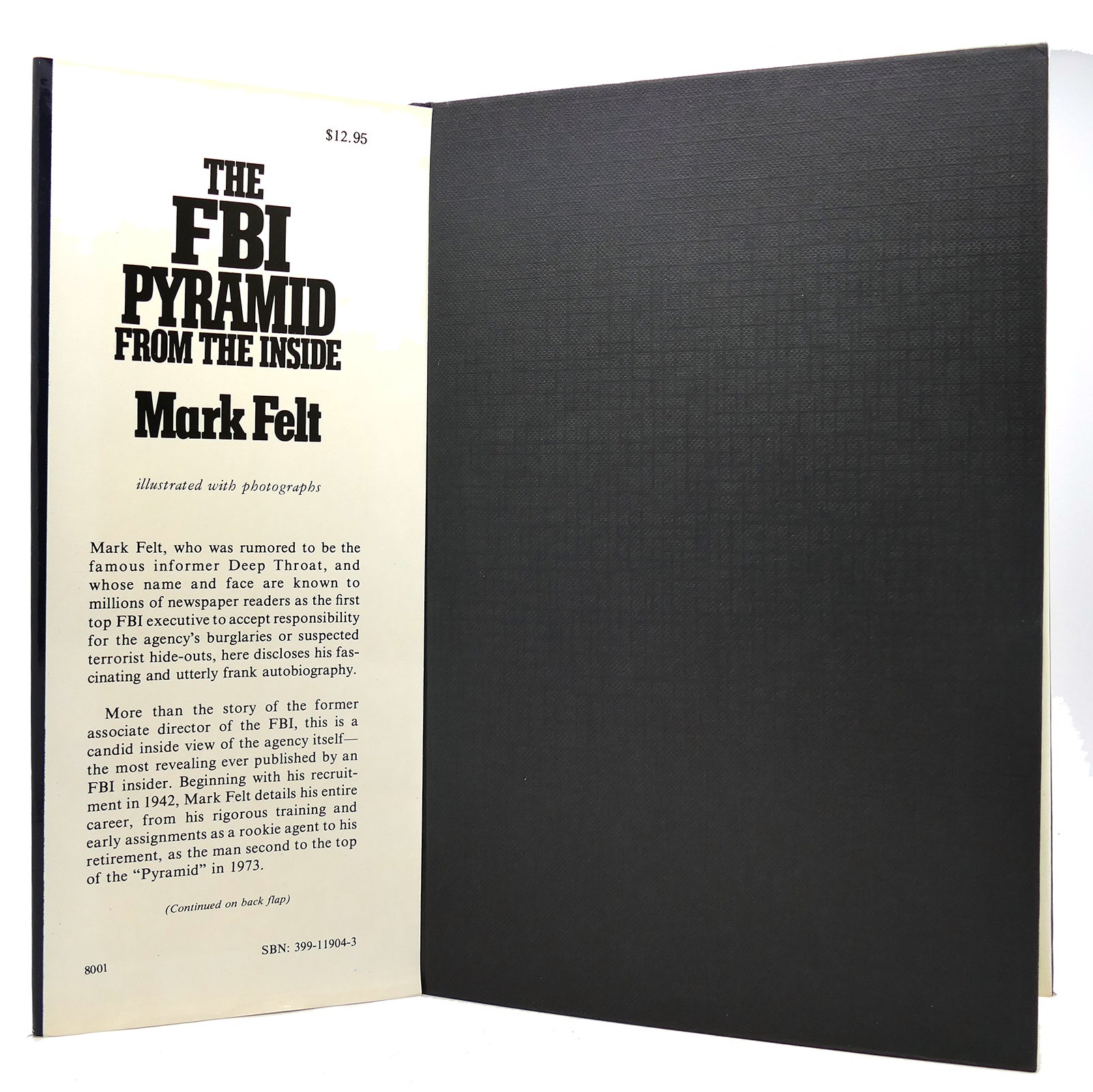The image depicts the inside dust jacket flap of a book. The book is slightly open, revealing its black front cover on the right and a folded-over dust jacket on the left. The dust jacket has a white background with black text. At the top, it displays the price, "$12.95." Beneath this, in bold text, it reads:

"The FBI Pyramid from the Inside"

The title is structured in such a way that each word is on a separate line, with "FBI" in smaller text that progressively enlarges, leading into the longer word "Pyramid." Below this is the author's name, "Mark Felt," followed by the phrase, "Illustrated with photographs."

The descriptive blurb underneath provides an insight into the book: "Mark Felt, who was rumored to be the famous informer Deep Throat and whose name and face are known to millions of newspaper readers as the first top FBI executive to accept responsibility for the agency's burglaries or suspected terrorist hideouts, here discloses his fascinating and utterly frank autobiography. More than the story of the former Associate Director of the FBI, this is a candid inside view of the agency itself—the most revealing ever published by an FBI insider. Beginning with his recruitment, Mark Felt details his entire career from his rigorous training and early assignments as a rookie agent to his retirement as the man second to the top of the 'pyramid' in 1973. Continued on back flap."

At the bottom of the flap, there are some numbers, including an SBN and the number 8001.